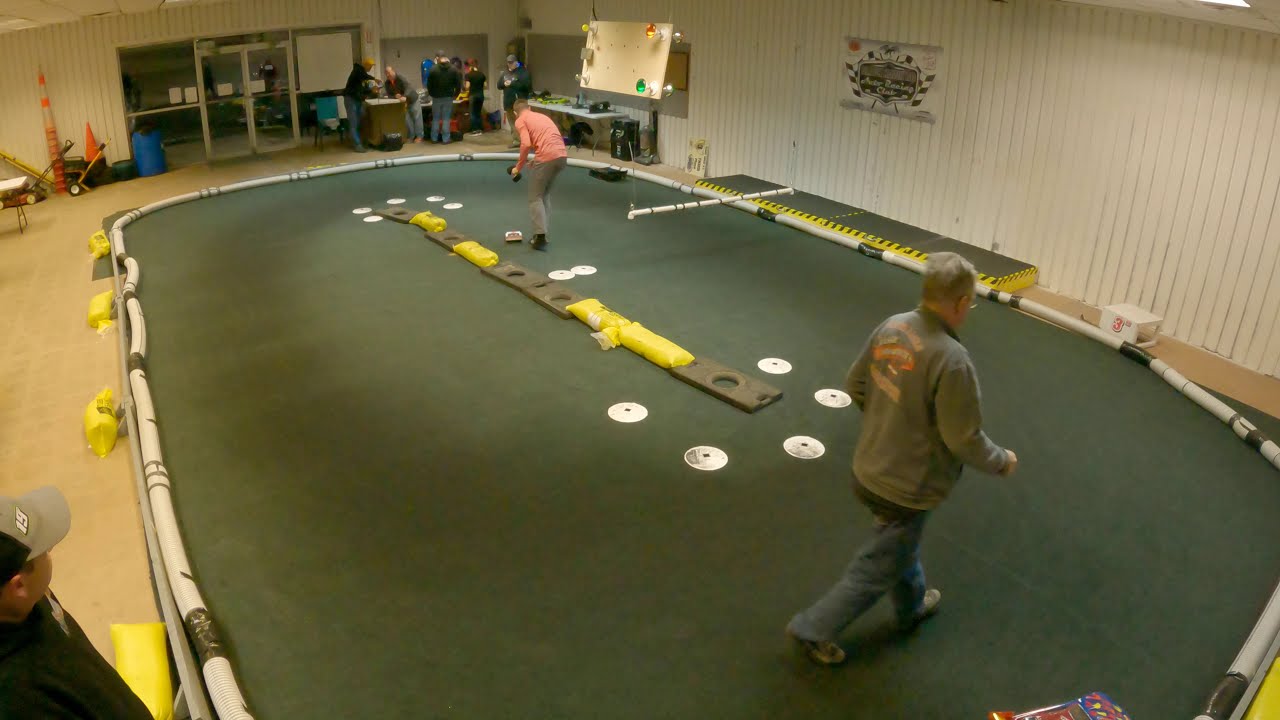The image depicts an indoor setting within a spacious metal building with white-boarded walls. The focal point of the scene is a large, green-carpeted area, around which foam tubes are arranged to create an oval-shaped track. Inside this track, various objects, including weights and yellow sandbags, are positioned, resembling the setup of a model racetrack. Situated within this space, there are several boards with holes aligned in a row, along with scattered discs or CDs.

Two men are actively engaged in arranging items on the green carpet. On the right, a man in a gray sweater and blue jeans walks purposefully, while another man in a pink shirt and gray pants bends over near the center, placing objects. In the background to the upper left, there are clusters of people milling about, some observing the setup and others seemingly involved in different tasks. Among them, a man in a gray and black cap and a black sweater stands out, watching the preparations from the lower left corner. A board with red, green, yellow, and white lights is also visible, implying some form of structured game or event, although its exact nature remains unclear.